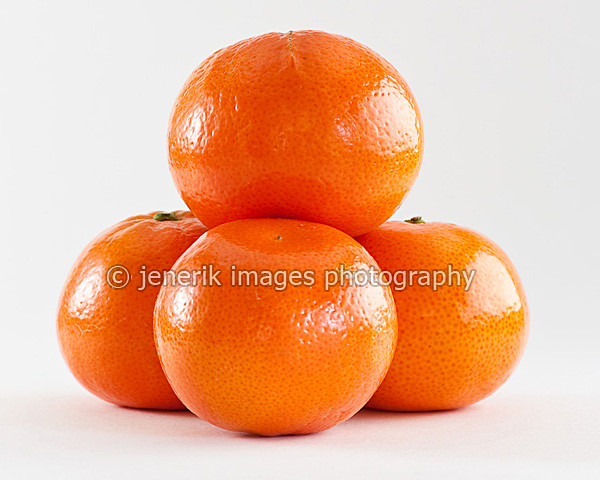This high-quality, color photograph captures four glossy, blemish-free oranges stacked in a pyramid formation against a pristine white background. Three oranges form the base, resting on a white surface with minimal shadows indicating their placement, while the fourth orange is balanced atop these three. The bottom-left and bottom-right oranges are positioned with their thick stems facing upwards, while the middle-bottom and top oranges have their thick stems facing downward. The image likely suggests the presence of a fifth, hidden orange supporting the structure from behind. Overlaid in ghosted white text across the middle of the photo, the copyright symbol "©" and the phrase "Jenerik Images Photography" is visible, with "Jenerik" uniquely spelled as J-E-N-E-R-I-K. The clementine-like oranges, highly reflective and possibly waxed, are arranged to highlight their striking appearance under professional lighting conditions.